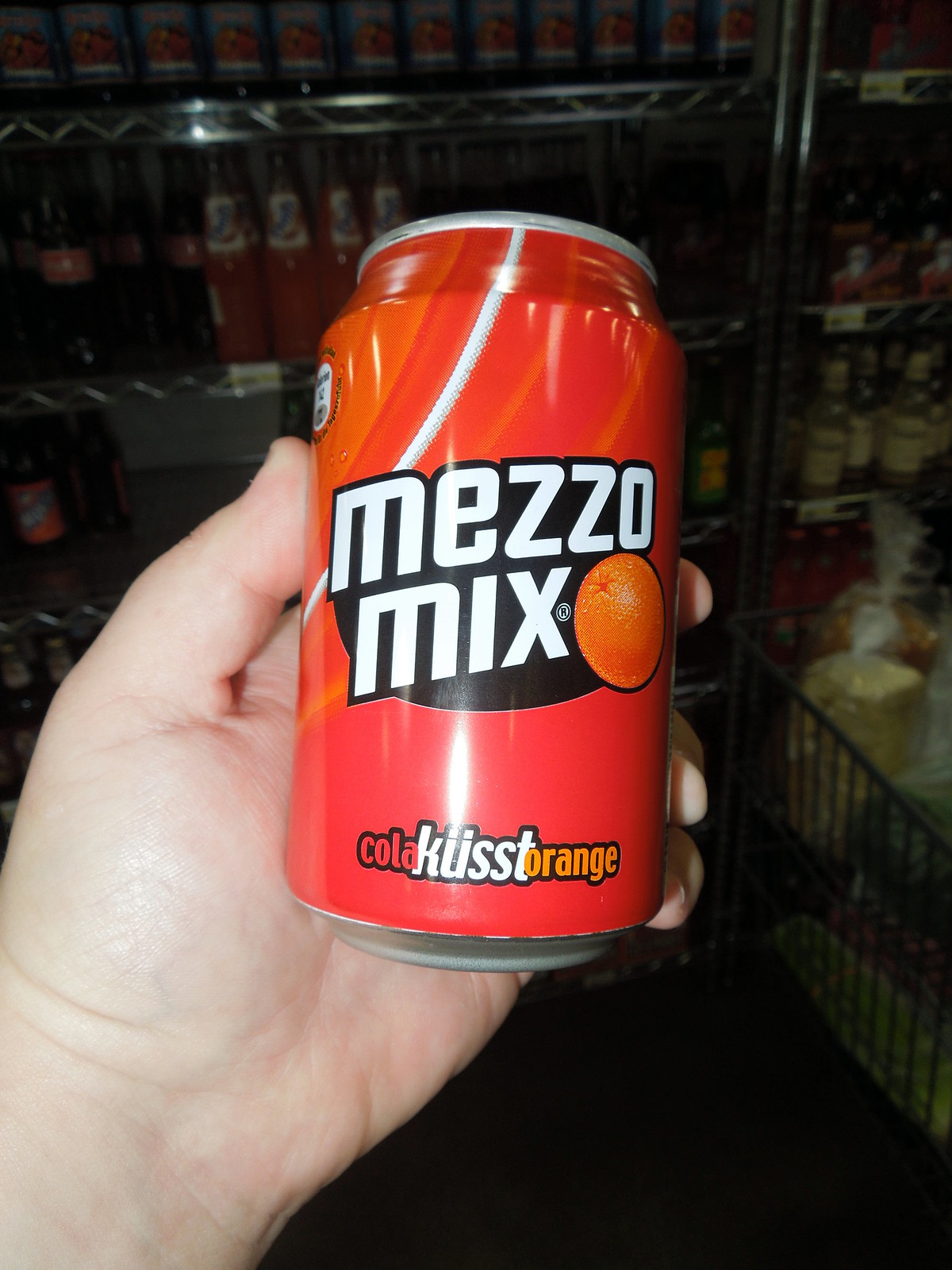In this photograph taken inside a grocery store or convenience store, the focus is on a can of Mezzo Mix soda held by a person's hand. The background showcases a gray floor and metal shelf racking stocked with an assortment of glass-bottled sodas, including recognizable brands like Coca-Cola and Fanta, along with various other sodas whose labels aren't legible. The hand entering from the bottom left belongs to a person with a paler skin tone, their palm facing upward with the thumb positioned on the left side of the can. The can itself features a gradient design transitioning from orange at the top left to red at the bottom right. Bold white text with a black outline spells out "Mezzo Mix," accompanied by an icon of an orange. Towards the bottom of the can, the text "Koloklist Orange," with "klist" spelled as K-L-I-S-S-T, is also visible in white print.